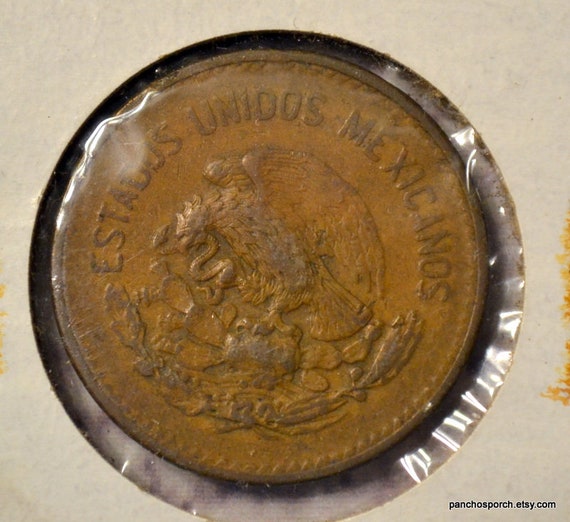This photograph showcases a bronze-colored coin, encased in a circular cardboard and plastic holder. The plastic covering makes the coin its centerpiece. Along the top edge of the coin, an inscription reads "Estados Unidos Mexicanos," which translates to the United States of Mexico. Central to the coin's design is an intricate emblem depicting an eagle perched atop a wreath-like structure, grasping a snake in its beak and talons. Surrounding the edge of the coin are rivet-like embellishments, complementing the silver rim that frames the coin. The outer white cardboard border is slightly stained brown and features the text "ponchosporch.etsy.com." This holder ensures the coin is well-preserved and clearly visible.